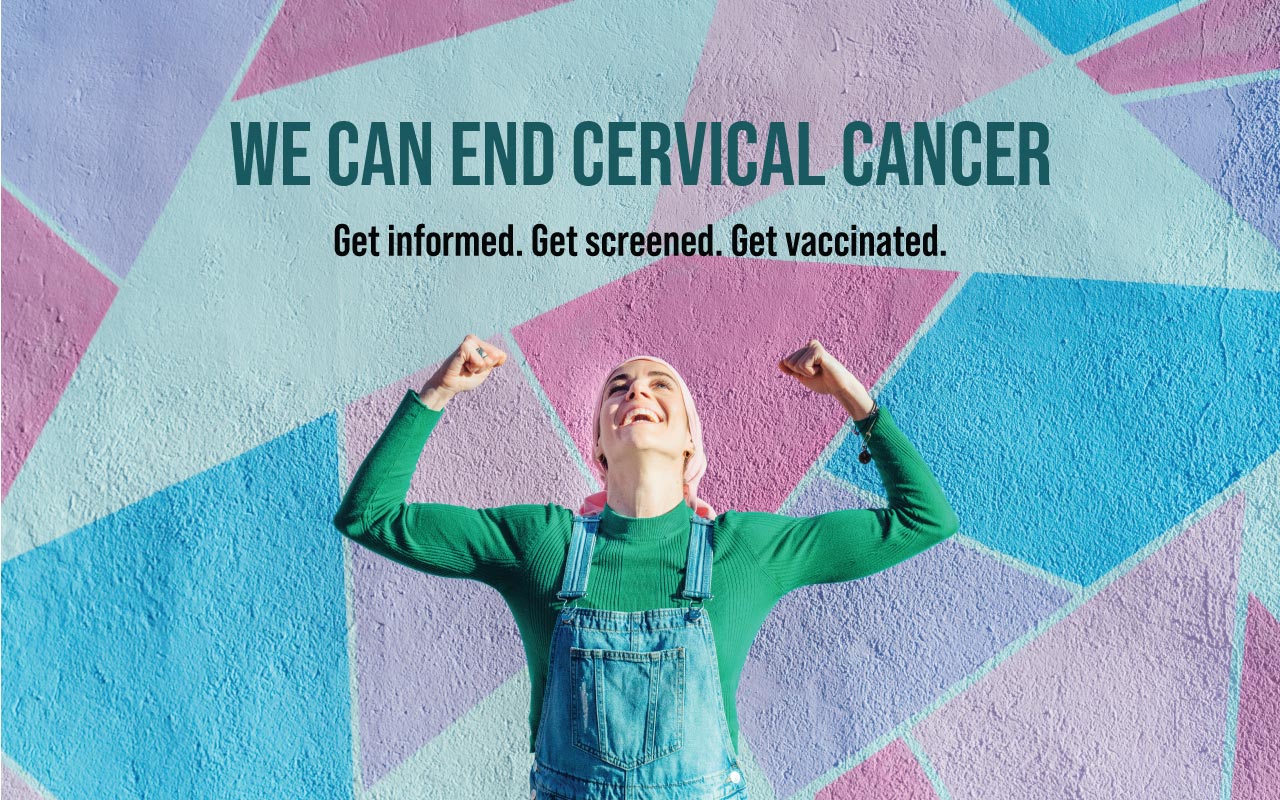The image is an infographic-style advertisement featuring a joyful woman standing straight against a colorfully painted cement wall adorned with pastel geometric triangles in blue, pink, purple, and off-white. She is dressed in blue denim overalls over a long-sleeved textured green turtleneck and has her hair wrapped in a pink head covering. With her fists raised in the air and her head thrown back in laughter, she looks up at bold, dark teal text that reads, “We Can End Cervical Cancer.” Below this, smaller black text encourages viewers to “Get Informed, Get Screened, Get Vaccinated.” Her expression radiates happiness and triumph, embodying the hopeful and empowering message of the advertisement.